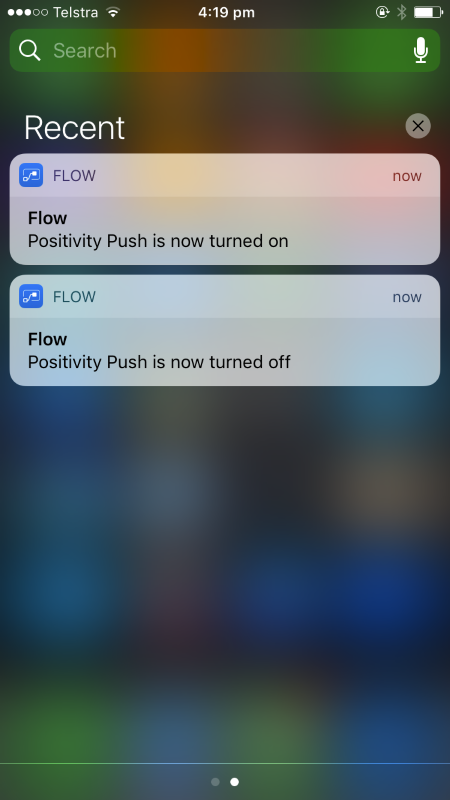The image depicts a tablet or a mobile phone interface with various elements displayed on the screen. In the top left-hand corner, there are three filled circles and two unfilled circles, indicating some form of selection or status icons. The screen shows the carrier name "Telstra" and confirms that Wi-Fi is in use. The time displayed is 4:19 p.m. and there is a lock icon enclosed in a circle with an arrow curving downward, likely indicating secure connection or screen lock status. The Bluetooth icon is active, and the battery is approximately 75% charged.

Towards the middle of the screen, there is a semi-transparent rectangle serving as a search bar. This bar has a white magnifying glass icon and the word "Search" in gray, alongside a white microphone icon, allowing users to either type or voice their search queries.

Below the search bar, the word "Recent" is displayed in white text. To the far right, there is a black 'X' inside a gray circle, suggesting an option to clear the recent activities or notifications. 

The interface shows two notifications from an app named "Flow." The first notification states, "Flow: Positivity push is now turned on." The second notification directly below it indicates, "Flow: Positivity push is now turned off." The Flow app icon is blue, featuring a small white square with a line leading into a filled white square.

At the bottom of the screen, there is a green line, which appears green due to the blurred, multicolored background consisting of blues, greens, browns, reds, and yellows. Additionally, there are two dots below this section, with the first dot unfilled and the second one filled, likely indicating the position within a set of pages or screens.